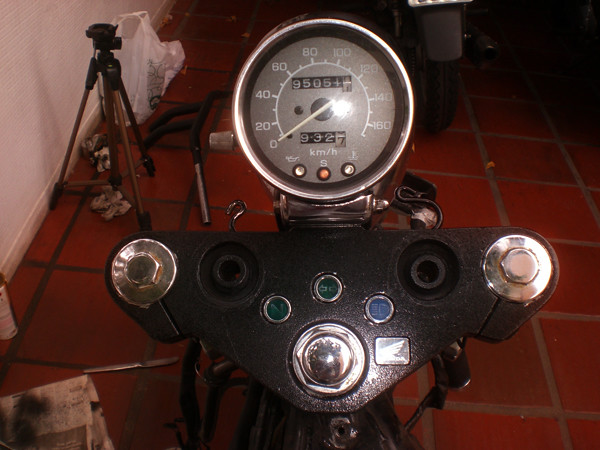This detailed photograph captures an analog motorcycle odometer, featuring a slate-colored dial with clear white numerals. The round chrome frame encloses the odometer, emphasizing its classic, vintage design. The odometer sits above the part of the motorcycle where handlebars would typically be attached, though they are currently missing. The scene appears to be in a workshop setting; the floor is covered in red tiles, and a camera tripod leans against the left-hand wall. Scattered below the motorcycle are newspapers speckled with dirt and fuzzy debris, hinting at recent cleaning activity. In the background, a figure is partially visible, identifiable only by their legs, which are clad in a gray coat and black pants, with black shoes completing their attire.